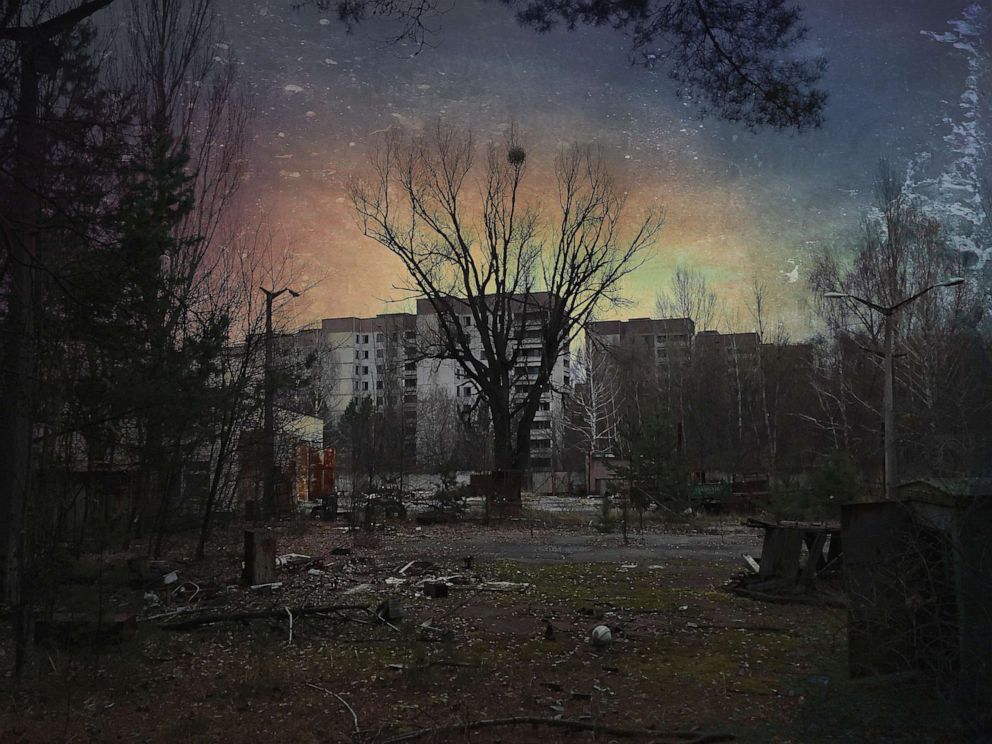The image depicts a gloomy, outdoor scene of an abandoned apartment complex set against a dark, dusky sky. The overall atmosphere is dreary and hazy, with visibility impaired by the lack of light. A faint orange hue in the sky suggests that the sun is setting. In the background, towering, dilapidated apartment buildings—approximately 8 to 10 stories tall—stand in silent decay. The structures are stark and white, contributing to the cold, neglected feel of the image. 

In the foreground, patches of overgrown grass are strewn with trash, adding to the scene's post-apocalyptic ambiance. A prominent tree, stripped of its leaves, stands lifelessly in the middle, while another leafless tree can be seen on the left. The overall scene is reminiscent of winter, with barren trees and a general sense of desolation permeating the image. Strewn along the ground are scattered pieces of debris, enhancing the impression of an area long abandoned and fallen into ruin. Despite a few streetlights, there is no sign of life or activity, and the lights remain off, casting the area in near-total darkness. The picture captures the forlorn beauty of a rundown urban landscape bathed in the muted colors of sunset.